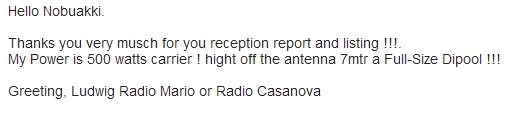In the image, a message is printed in black text on a white background. The text reads:

"Hello, NOBUAKI.  
THANKS YOU VERY MUCH FOR YOUR RECEPTION REPORT AND LISTING!!!  
My power is 500 watts carrier! Height off the antenna 7 meter, a full-size dipole!!!  
Greeting, Lyric Radio Mario Casanova."

This appears to be an informal communication, possibly resembling an email or a letter, with multiple typos and grammatical errors.